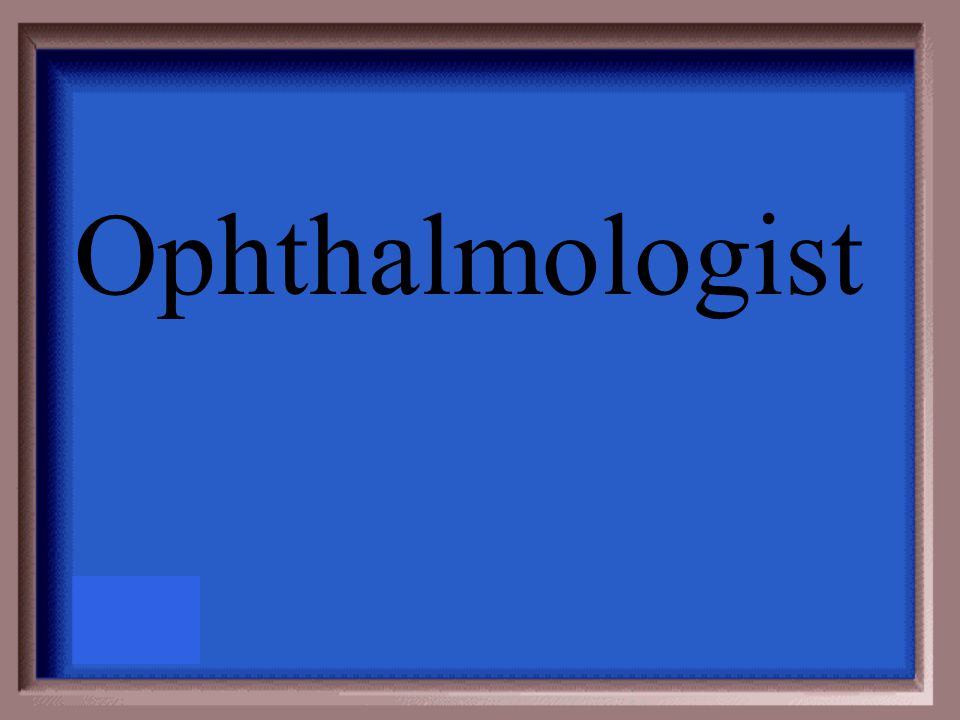The image depicts a plain, computer-generated sign that could be used in a doctor's office. It features a rectangular, medium-brown wooden frame with varying shades of color. The inner border shifts from a darker brown on the upper portion and left side to a white hue on the right and bottom edges. Within this frame is a solid, bright blue background. Horizontally centered towards the upper part of this blue space is the word "Ophthalmologist" printed in plain black text, with a capital "O." The image is simple and devoid of any other objects, images, or additional text. The design suggests it might be a template or placeholder for a professional sign, possibly indicating a job title.